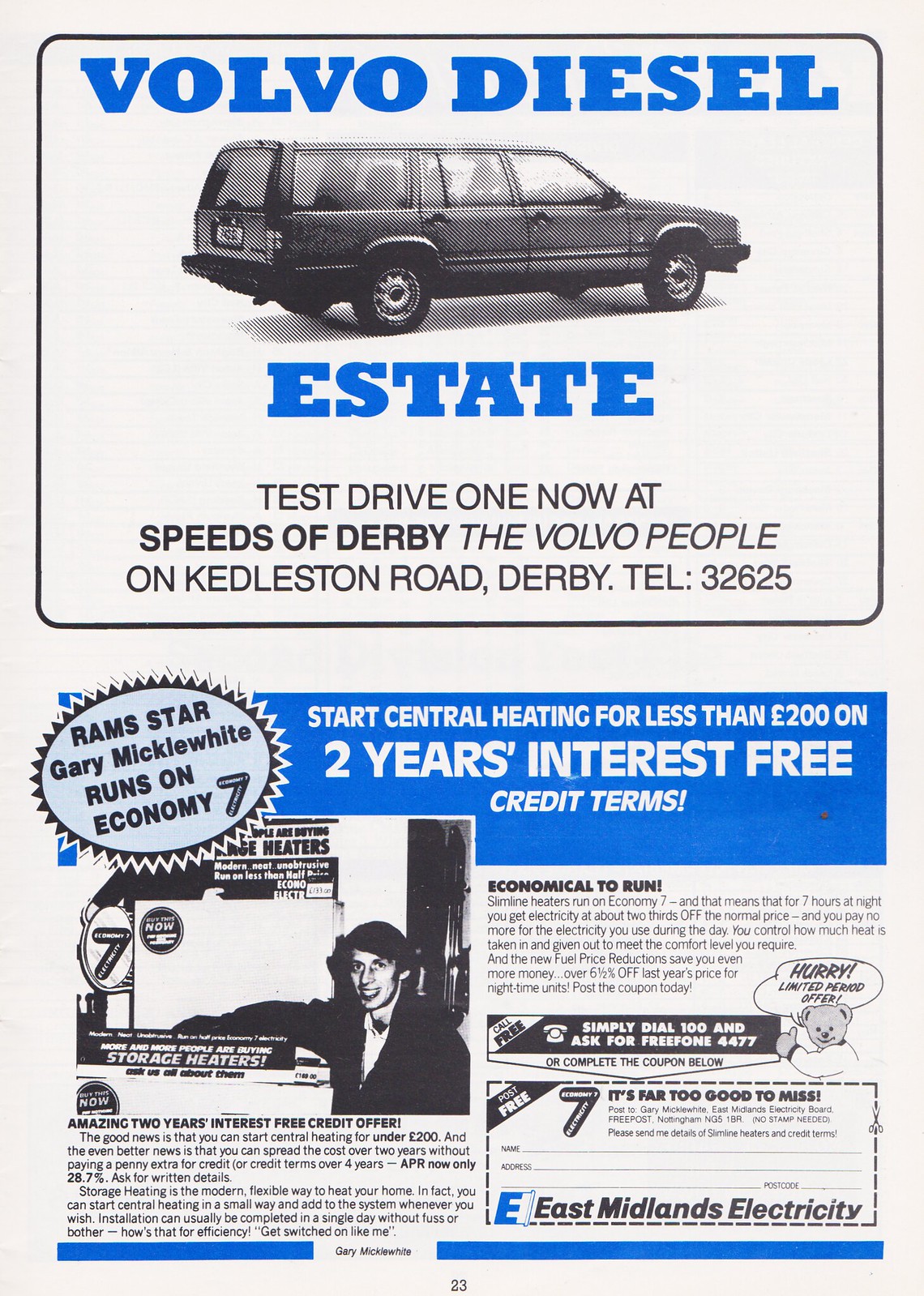This page, printed in blue and black ink on white paper, appears to be from a program or magazine, specifically page 23. It features two distinct advertisements. The top half promotes a Volvo Diesel Estate. The headline "Volvo Diesel Estate" is prominently displayed in blue text, with a black and white image of an old Volvo station wagon placed between the words "Volvo Diesel" and "Estate." Below the car image, in black lettering, it reads: "Test drive one now at speeds of Derby, The Volvo People on Kedleston Road, Derby, Tel: 32625." 

The bottom half of the page advertises an economical heating solution by East Midlands Electricity. It boasts a large blue banner across the top with white text announcing: "Start central heating for less than 200 euros on two years interest-free credit terms." A light blue circular burst on the top left corner features a black and white photo of soccer player Gary Micklewhite with the caption: "Ram star Gary Micklewhite runs on Economy 7." The ad highlights an amazing two-year interest-free credit offer for slimline heaters and states the affordability of starting central heating. It includes a postal form at the bottom right for potential customers to fill out their name, address, and postcode, emphasizing a "far too good to miss" promotion.